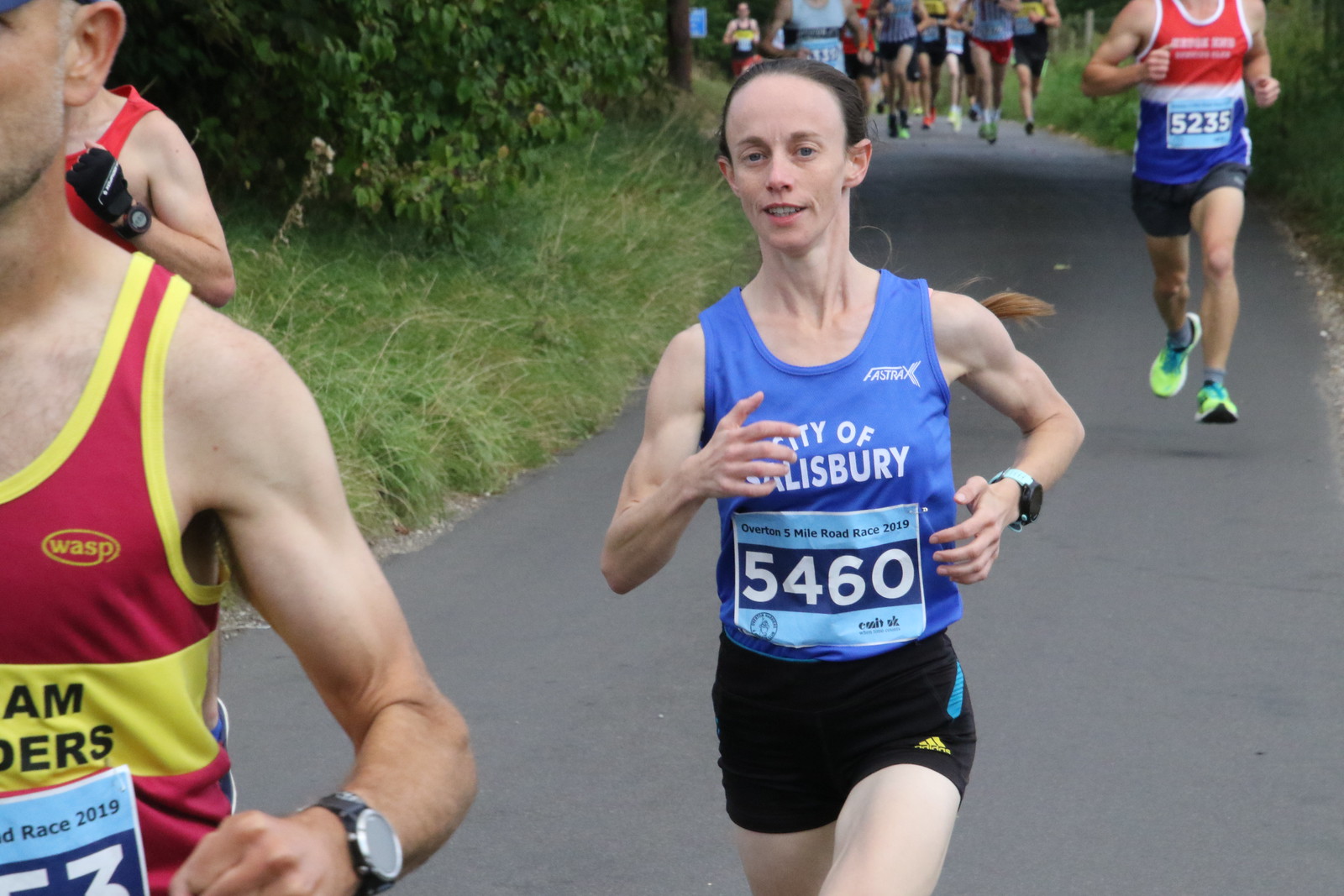The image captures a bustling scene of a road race taking place on a paved asphalt path, likely within a park given the greenery and foliage on both sides. Dominating the center of the image is a prominent runner, a young man in mid-stride, wearing a blue jersey emblazoned with "City of Salisbury" in white letters, black Adidas shorts, and a watch. His race number, 5460, is affixed to his shirt with a stick pin, and the number patch bears the additional details of "Overton 5 Mile Road Race 2019" and "EMITUK." 

Behind him, another runner is visible, clad in a red, white, and blue jersey with the number 5235 and green running shoes, though their face is not discernible. Further in the background, another runner can be seen wearing a red jersey with yellow accents, though their race number is obscured. Surrounding these key figures, a larger group of runners follows in pursuit. The lush greenery flanking the path indicates it is a summer day, lending a vibrant and energetic backdrop to the athletic endeavor.